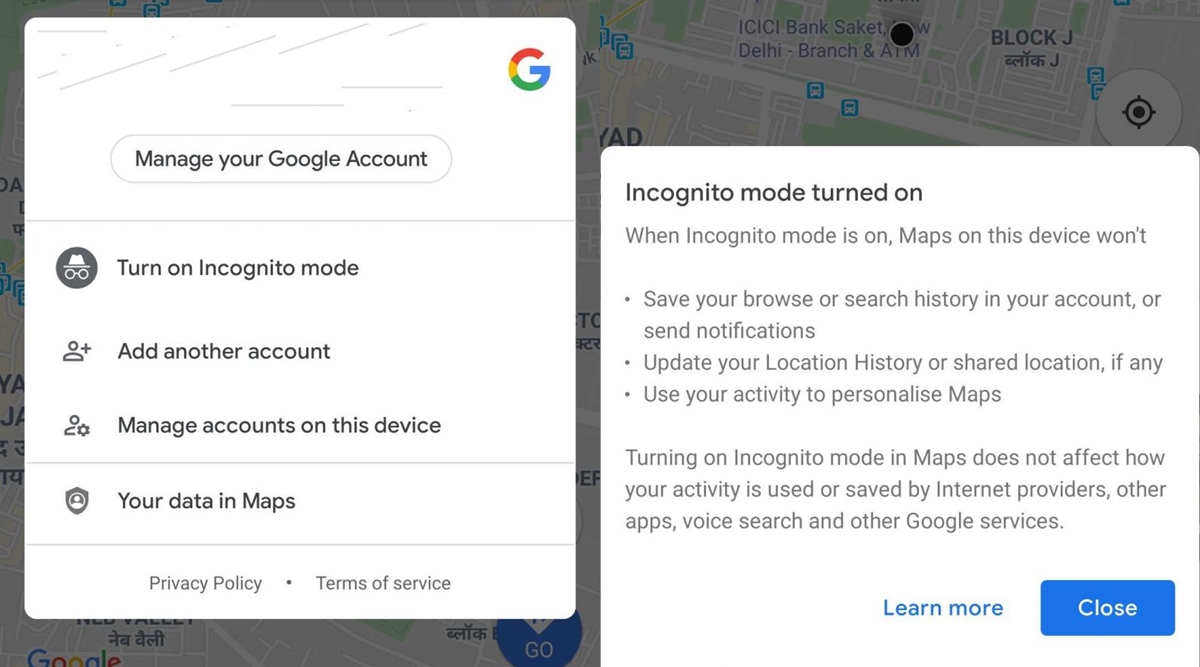In the background of the image, a Google Maps interface is visible, displaying various roads labeled with names, alongside a few distinctive blue location markers. On the left side of the screen, a white pop-up box appears, featuring the Google "G" logo in its characteristic red, yellow, green, and blue colors at the top right corner. The box is structured into several distinct sections separated by fine gray lines.

The first section is headed by the text "Manage your Google Account." Below this, it offers options to "Turn on Incognito mode," accompanied by the incognito icon, a black circle with a white hat and glasses. Followed by options to "Add another account," and "Manage accounts on this device." The next section bears the title "Your data in Maps," illustrated with the Maps icon.

Further down, it provides links to the "Privacy Policy" and "Terms of Service."

On the right side of the screen, another pop-up message is visible, headed with "Incognito mode turned on." The message explains the implications of using incognito mode in Maps: it won't save your browsing or search history, send notifications, update your location history, or use your activity to personalize Maps. It also clarifies that turning on incognito mode in Maps won't affect how your activity is used or saved by internet providers, other apps, voice search, and other Google services.

At the bottom of this pop-up, in blue text, are options to "Learn more," and a blue button labeled "Close" in white text, allowing users to dismiss this informational screen.